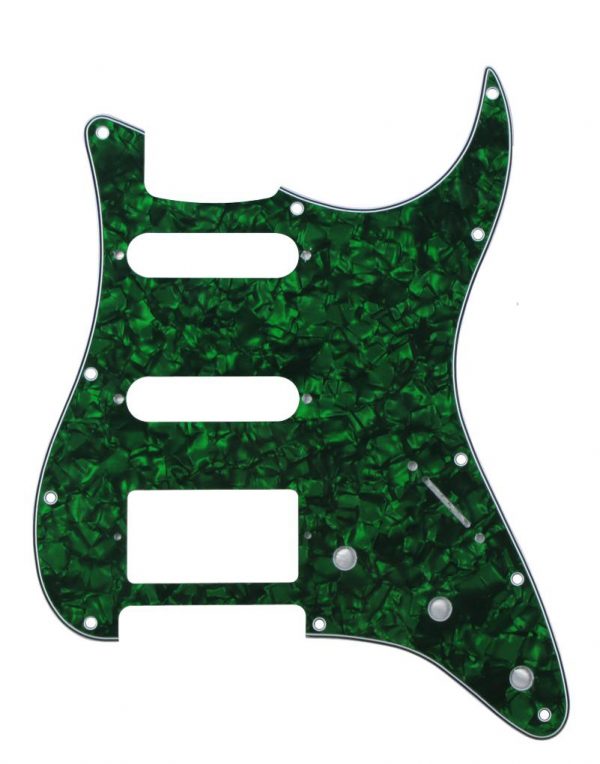In the center of a completely bright white background lies an object resembling the base part of a guitar without any strings or a stem, akin to a guitar shell. Dark green, resembling green grass or pebbles, forms the primary background of this shell, with details accentuated by cutouts revealing the white background. These cutouts consist of thin ovals at the top and a larger rectangle toward the bottom. Small white and light gray circles near these cutouts appear to imitate bolt positions for attaching the guitar face. The object also features floral patterns and has a scattering of twelve small holes around it, and three silver buttons arranged diagonally. Additional shapes, including two octagons and two squares, contribute to the intricate design. The overall color palette includes dominant dark green with hints of black, white, and gray. The vignetted object is centered, giving the impression of a detailed, well-crafted component, possibly a purposeful tool or a decorative overlay suitable for a guitar or multi-functional item.